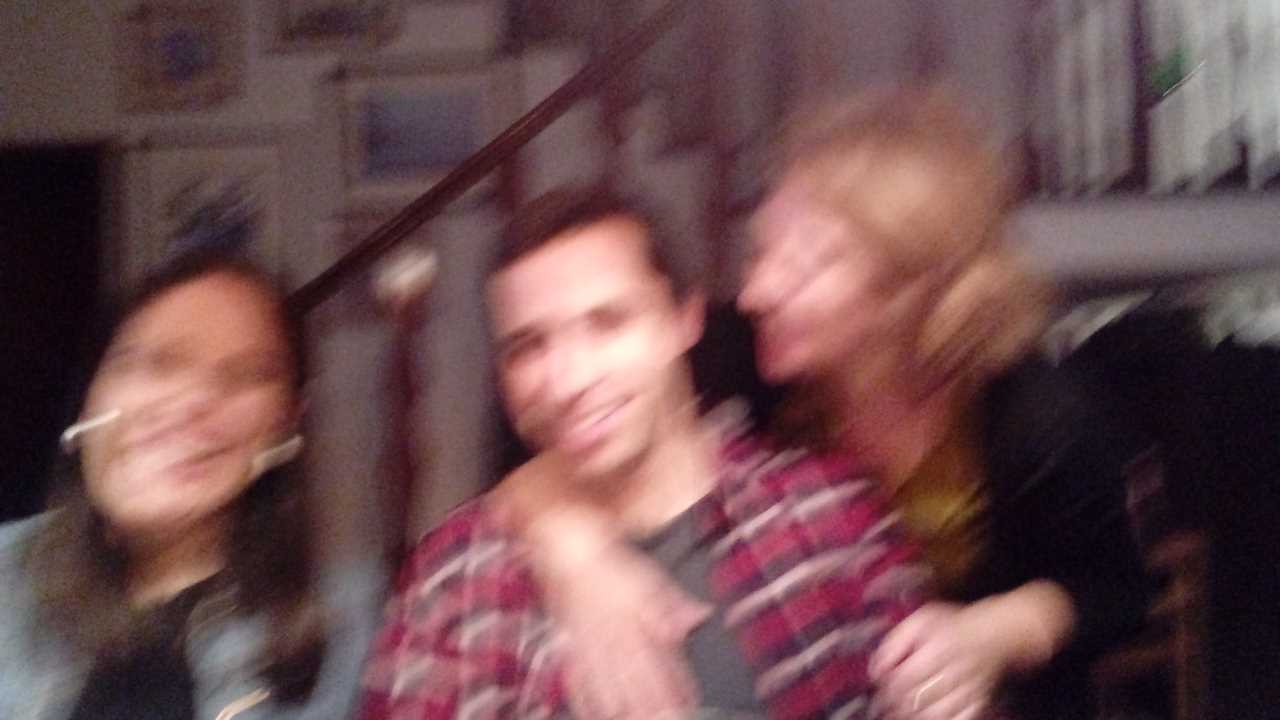In this slightly blurry color photograph taken inside a home, three individuals are seen gathered around a table, with a staircase visible in the background. The staircase starts on the left side of the image and ascends towards the right. Along the wall opposite the staircase, several framed pictures are hung. 

At the center of the group sits a man wearing a gray shirt layered with a red plaid shirt. To his left stands a woman with long brown hair, adorned with earrings, dressed in a black shirt and a gray jacket. On his right, a blonde woman in a gold shirt and black sweater is leaning over him, her right arm draped over his right shoulder, as if whispering something into his ear. The intimate and candid nature of the scene, coupled with the soft blur of the image, adds a warm, homey charm to the photograph.